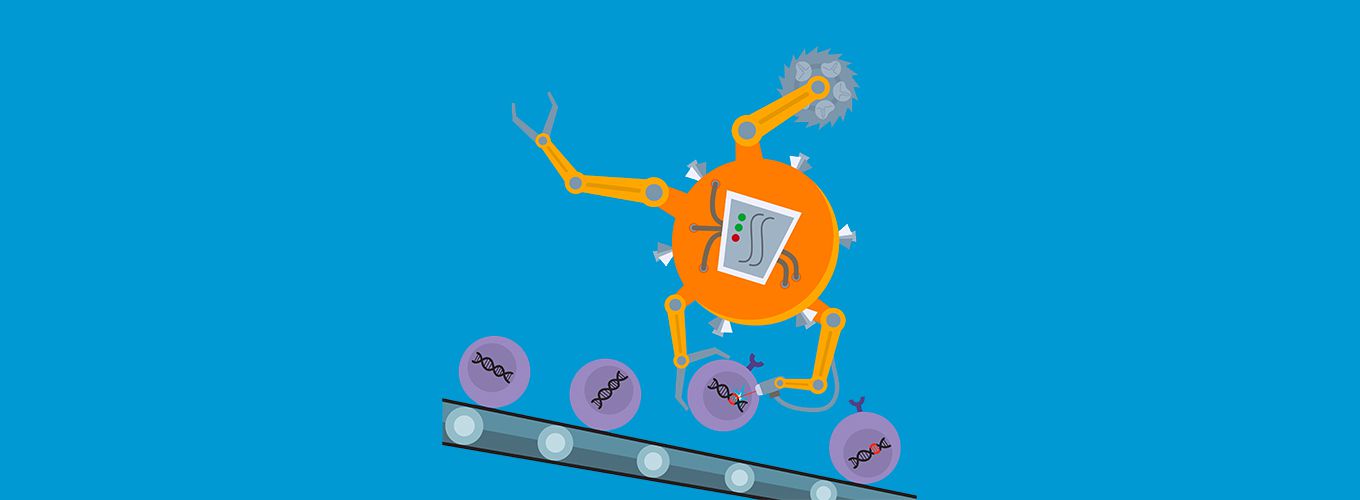In a horizontal rectangular frame with a deep teal-blue background, an animated industrial robot dominates the scene. The robot, spherical and orange in color, is suspended above by a jointed attachment and adorned with six white spikes around its circumference. Below, it has several jointed appendages resembling mechanical arms and legs, each equipped with different tools: pinchers, circular saw blades, and more. One arm, a smaller appendage attached to the bottom of its circular body, holds a circular, purple object lined with a genetic double-helix pattern. This object is one of four similar ones traveling on a side-view conveyor belt, distinguished by the rollers at each end. The robot manipulates these objects with precision, suggesting a bustling, automated assembly line at work.